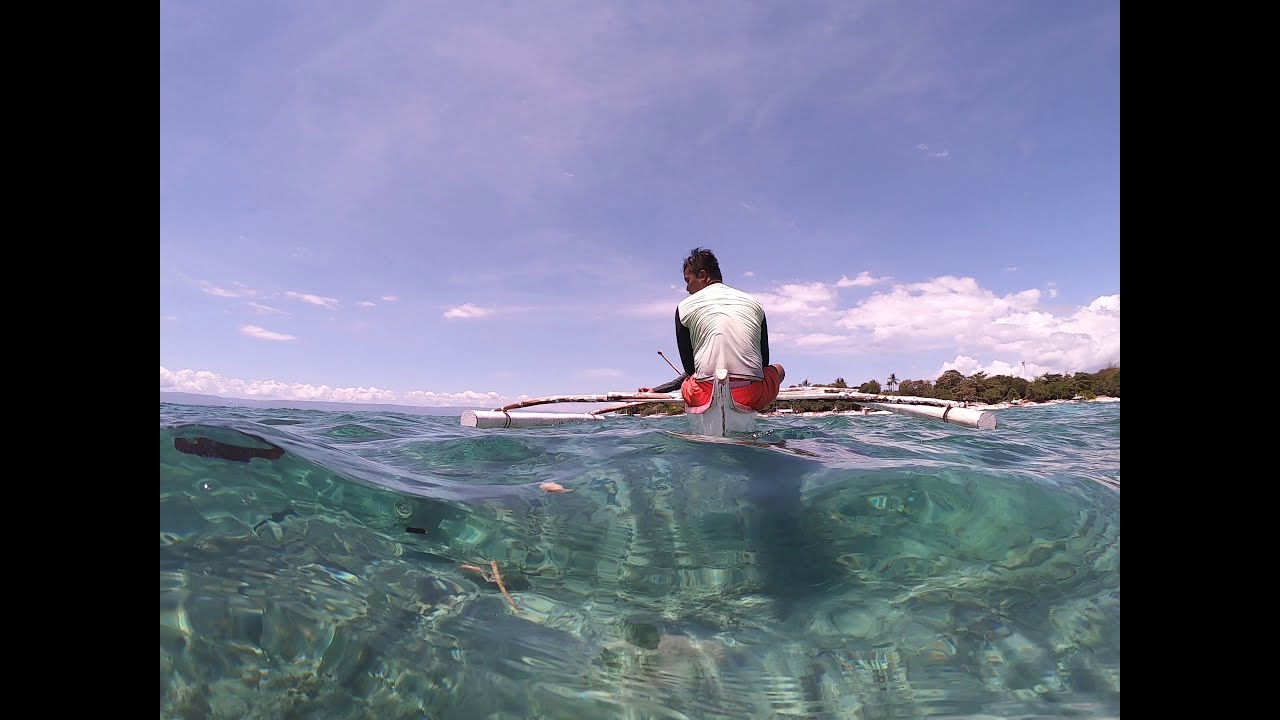In the image, there appears to be a man on some sort of canoe-like boat, equipped with flotation stabilizers on each side, making it resemble a surfboard or kayak hybrid. The water, very clear and light aqua in color, is almost level with the camera, giving the impression that the camera is partially submerged. The man is positioned with his back to the viewer, wearing a white shirt with dark sleeves and red shorts. He has dark hair, and you can see the profile of his face. On his left in the water, there is a dark object vaguely resembling a fish. In the distance, the horizon is filled with trees and palm trees, and the sky above is a vibrant blue with patches of clouds and a fog bank to the far left. The scene captures a serene moment on what seems like a warm, sunny day in the middle of the ocean, with a distinct view of both the aquatic foreground and the verdant shoreline in the background.